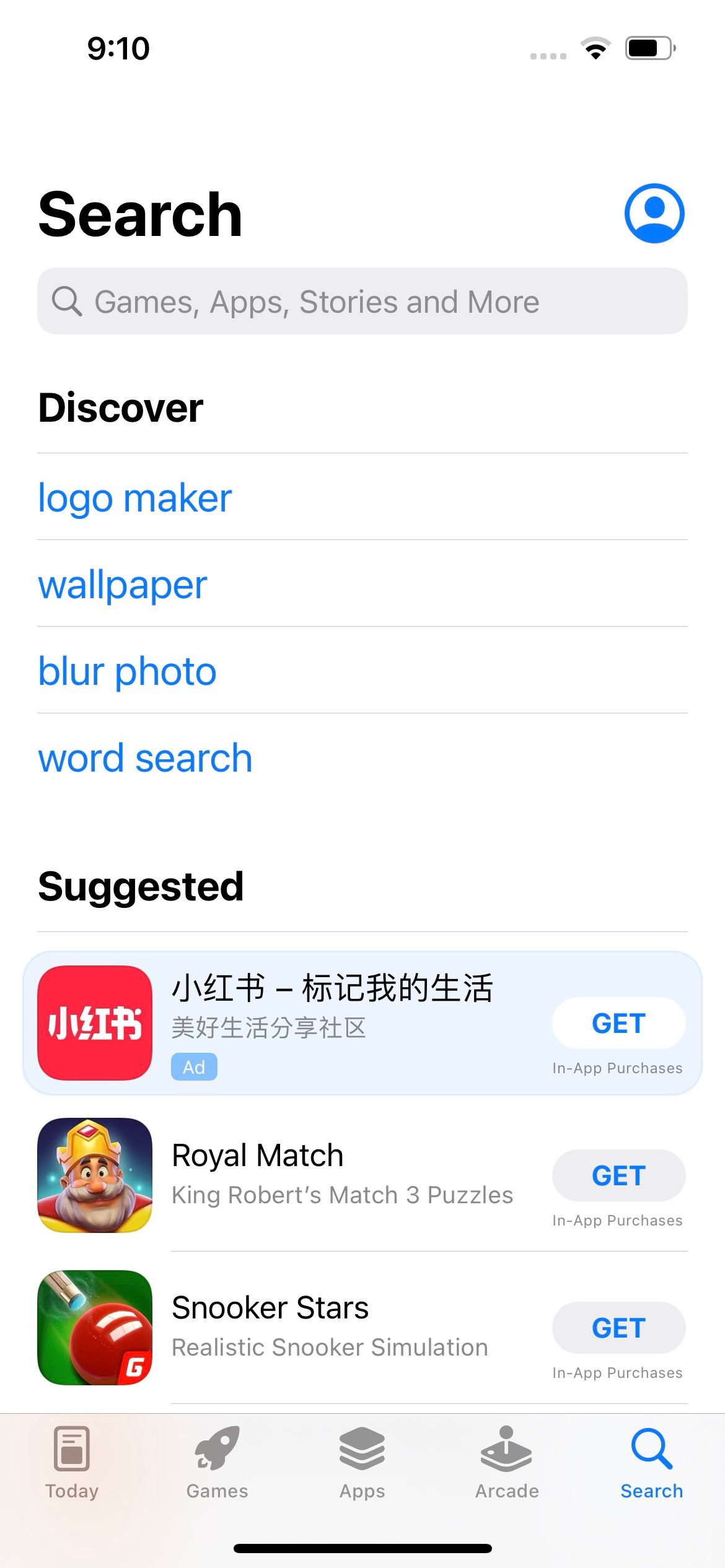**Screenshot of a Mobile App Store Search Page**

This screenshot, taken on a cell phone at 9:10 (as indicated by the time display at the top), shows the Wi-Fi and battery icons. The bold black text 'Search' is displayed at the top left, adjacent to a blue circle containing a blue silhouette of a person on the right.

Beneath this is a gray search bar featuring a magnifying glass icon and the placeholder text 'games, apps, stories, and more'. Below the search bar are tab categories such as 'Discover', 'Logo Maker', 'Wallpaper', 'Blur Photo', 'Word Search', and 'Suggested'.

The main section of the screenshot displays several app ads and suggestions. On the left, there is a red square with Asian lettering inside, accompanied by more Asian characters to the right. Below this, it says 'Add', 'Get', and 'In-App Purchases'.

Further down, there is an image showing a square cartoon of a man with a crown, mustache, and full beard, labeled 'Royal Match: King Robert's Match Three Puzzles' followed by 'Get' and 'In-App Purchases'.

Next to this, another app is showcased with a square graphic depicting a red billiard ball and a cue stick poised in the top left corner, labeled 'Snooker Stars: Realistic Snooker Simulation', followed by 'Get' and 'In-App Purchases'.

At the bottom of the screenshot is a menu bar with tabs labeled 'Today', 'Games', 'Apps', 'Arcade', and 'Search'. The 'Search' tab is highlighted, indicating the current section being viewed.